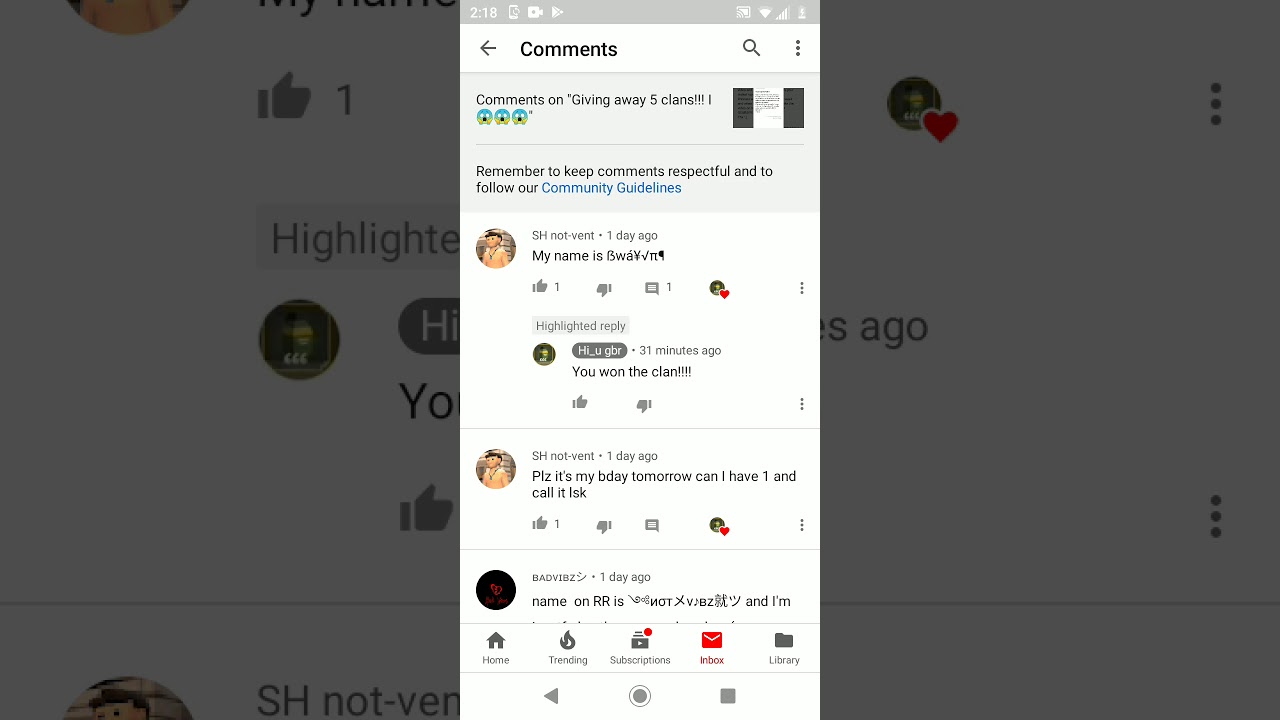This image is a detailed screenshot of a YouTube comment section, viewed on a mobile phone. The screenshot captures a zoomed-in and darkened background, giving prominence to the comment section that appears as a central pop-up display.

At the top left, the time is shown as 2:18, and the top right features an icon indicating the phone's battery is charging, denoted by a lightning bolt symbol. Centered at the top of the screenshot is the heading "Comments." Directly beneath this, a subheading reads "Comments on giving away five clans," presumably the video title, which includes the word "I" followed by three scared-face emojis. Directly underneath, a reminder prompts viewers to "remember to keep comments respectful and to follow our community guidelines."

The primary focus of the screenshot is a comment by a user named "shnotvent," stating, "my name is Bwav." Below this, a reply from the video creator, identified as "hi you goober," announces, "you won the clan." This indicates that "Bwav" is the recipient of one of the clans being given away in the video.

Further down, another comment from "shnotvent" reads, "please, it's my birthday tomorrow, can I have one, and call it, I guess, kay?" indicating a request for another clan. This detailed snapshot effectively conveys the context and interactions within the YouTube comment section surrounding a giveaway event.